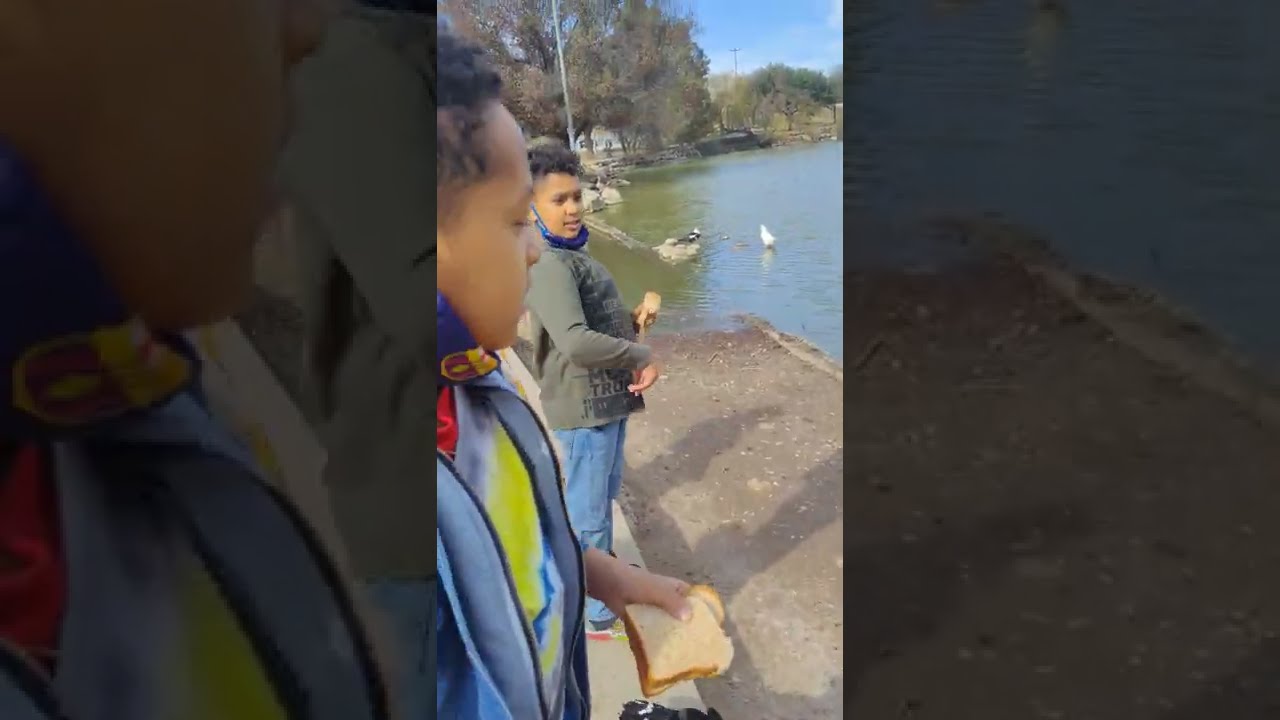The image shows two young boys standing by the edge of a lake, casually feeding birds with pieces of bread. They both have dark brown skin and are wearing long-sleeved jackets along with blue masks that hang below their chins, suggesting it was taken during the COVID-19 pandemic. The boys appear to be enjoying a day of outdoor recreation. One boy gazes out at the water while the other looks in a different direction, possibly at the birds. The scene is set against a background of blue sky with a few clouds, an assortment of trees, and a bridge. There are additional elements such as telephone poles, a house, rocks, and more birds perched on the rocks. The colors in the photo include shades of brown, black, white, green, gray, blue, red, yellow, and a hint of orange. The body of water looks typical for a lake, not overly clean but not terrible, and both boys are standing on a concrete or dirt surface near the water’s edge.